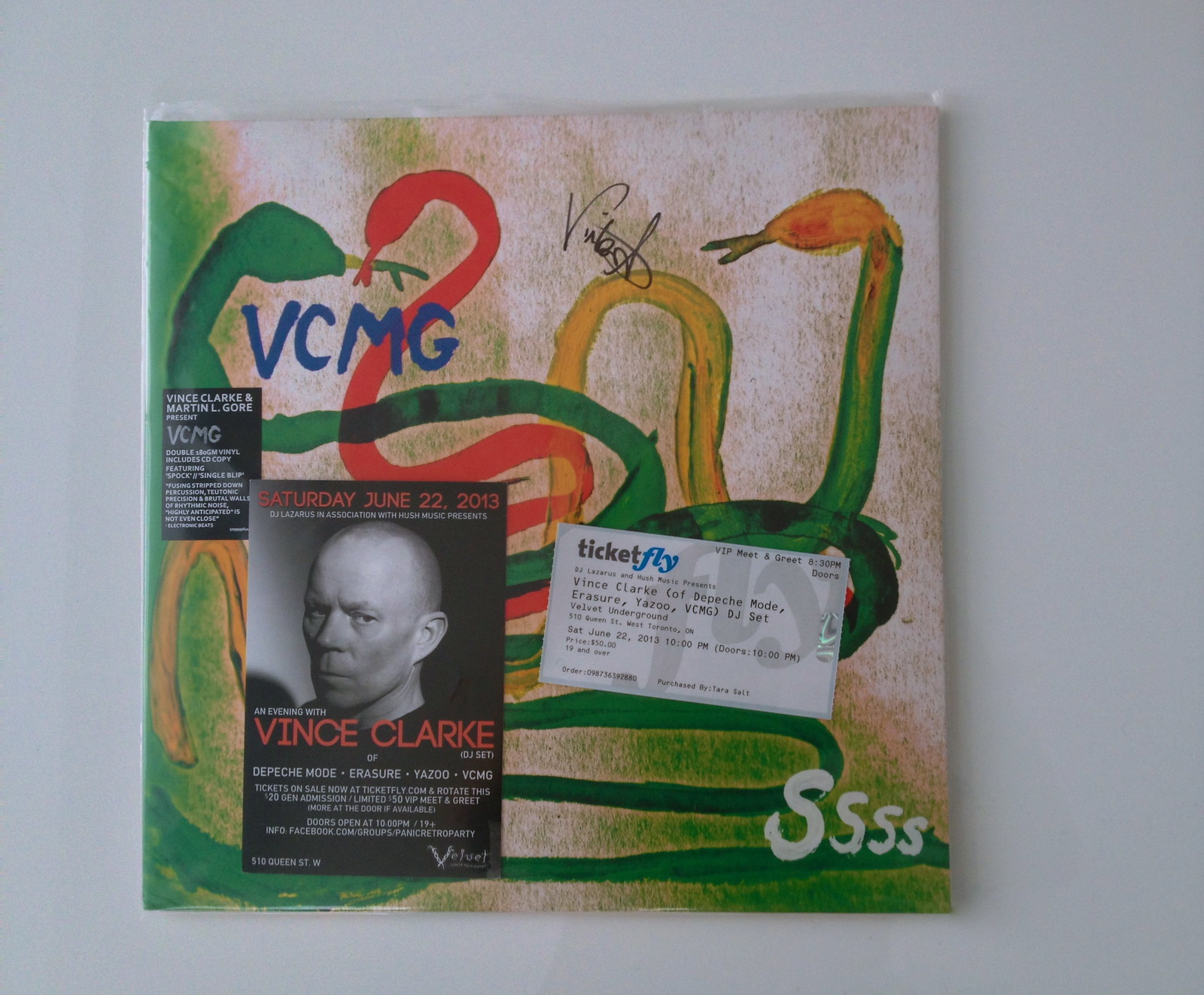The image is a photograph, likely of a vinyl album cover or a promotional flyer, featuring intricate painted artwork. The dominant image comprises a few abstract, colorful birds or snakes. Specifically, there is a green one, a red one, and another that transitions from yellow to green to orange. These figures are set against a background of mottled greens and beiges. In the bottom right-hand corner of the artwork, the letters "SSSS" are inscribed, which may suggest a hissing sound.

Accompanying the artwork are several printed materials. A prominent brochure states, "Saturday, June 22nd, 2013," advertising an event featuring Vince Clarke of Depeche Mode, Erasure, Yazoo, and VCMG. It mentions that tickets are available on Ticketfly, with options for general admission and VIP meet and greet passes. The text hints at further information available on Facebook.

Additionally, there is a black and white photograph of a man, presumably Vince Clarke, with a stern expression, a shaved head, and wearing a dark shirt. This image, along with other small text and details about the event, is printed on a white background with colors including black, white, red, orange, yellow, green, off-white, and tan.